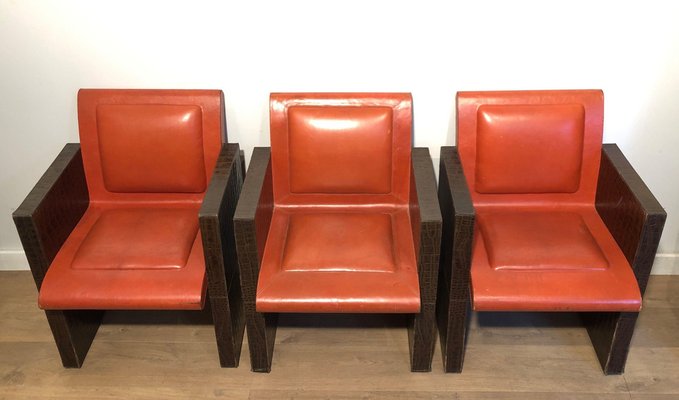The image showcases three identical chairs, aligned in a row from left to right, centered in the photograph. Each chair features a sleek design with dark wooden armrests composed of simple, vertical rectangular blocks that extend from the top down to the floor. The seats and backs are adorned with striking red cushions, which appear shiny, suggesting an indoor setting with a glare from a light source behind the photographer. The seats are flat with minimal, slightly raised cushioning, providing a streamlined appearance. The background consists of a stark white wall, and the chairs are placed on a light tan hardwood floor, further emphasizing the clean and modern aesthetic of the scene.